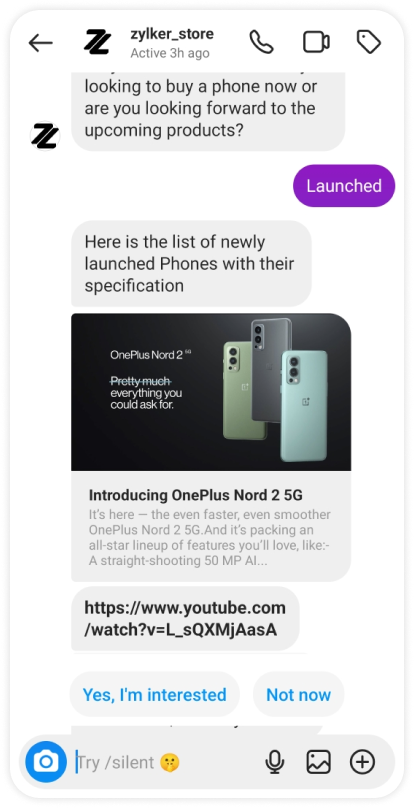This image is a detailed screenshot captured in portrait mode. The background is entirely white, and the content is presented in a single, elongated column. 

In the upper left-hand corner, there is a black back arrow followed by a unique logo resembling a combination of a numeral '7' and a sideways 'L', creating an appearance similar to the letter 'Z'. Next to the logo, the store's name "Z-Y-L-K-E-R_store" is displayed, along with the status "active three hours ago."

In the upper right-hand corner, there are icons depicting a phone and a possible price tag. Below, a message from the Zykler Store is shown on a gray background, reading: "Looking to buy a phone now, or are you looking forward to the upcoming products?" The recipient's response on the right-hand side states: "Launched."

Following the response, the Zykler Store replies with: "Here is the list of newly launched phones with their specifications." Below this message, set against a black background, is an advertisement for the "OnePlus Nord 2." This section includes an image showing three phones in light green, silver, and aqua colors, accompanied by the text: "OnePlus Nord 2, pretty much everything you could ask for."

Beneath this, there is further information introducing the "OnePlus Nord 2 5G." The description reads: "It's here, the even faster, even smoother OnePlus Nord 2 5G, and it's packing an all-star lineup, features you'll love." Directly underneath this text is a YouTube link. At the bottom of the screenshot, there are two buttons: a blue button on the left labeled "Yes, I'm interested," and a button on the right labeled "Not now."